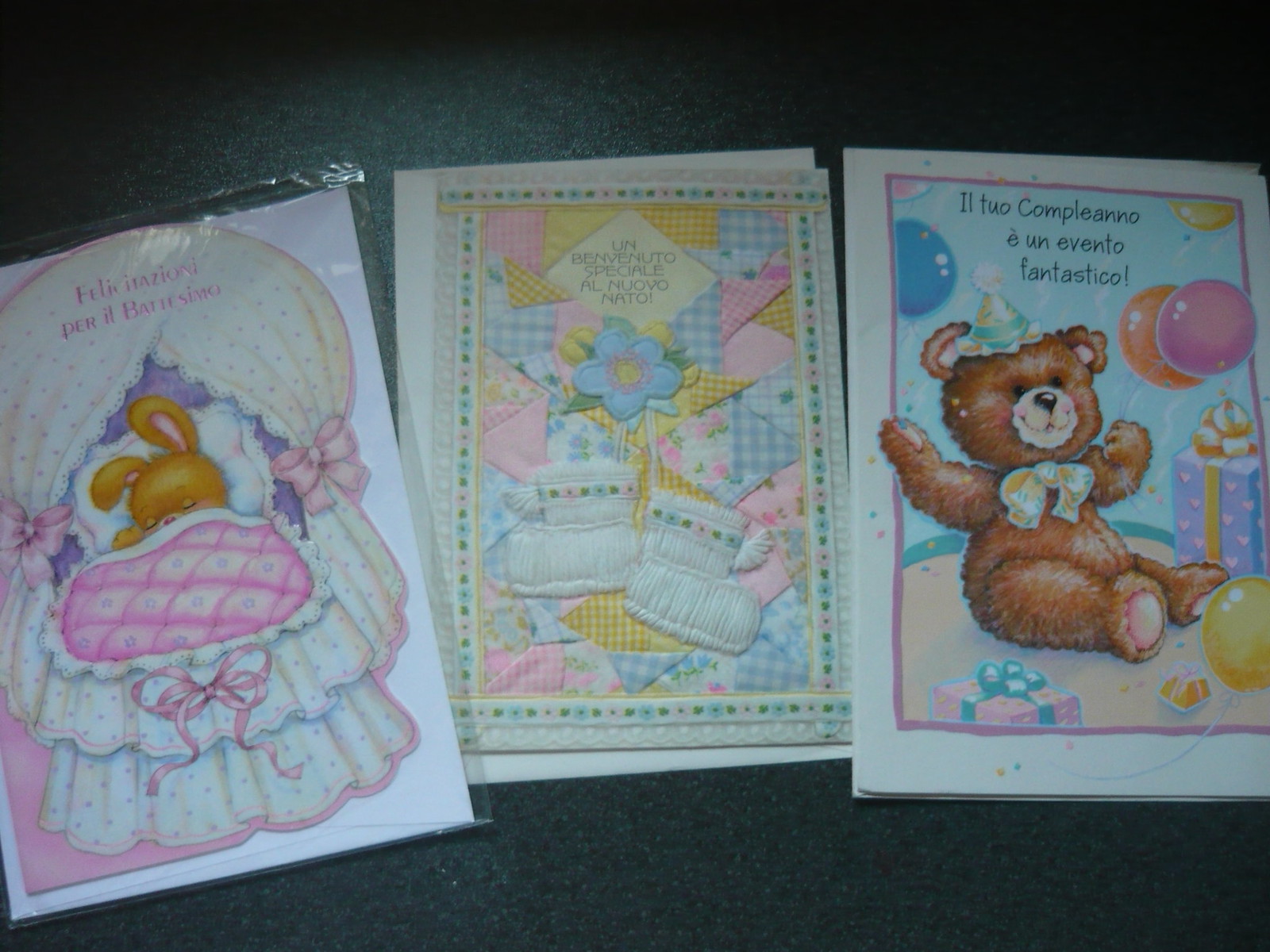This image captures three distinct greeting cards, each designed for different baby-related occasions, against a dark, likely gray, desk backdrop. The first card on the left presents a cozy scene of a small golden rabbit nestled in a bed, covered by a pink blanket. Surrounding its head is a white cloth material, and the card is adorned with Spanish text at the top. The central card features a tactile 3D design with a pair of white baby boots, surrounded by a colorful quilted pattern of blues, pinks, and greens. The text "Un Benevuto Special Añojo Nato" is prominently displayed in the middle. The third card on the right showcases a joyful brown teddy bear wearing a party hat and a ribbon around its neck. The bear is surrounded by balloons in blue, orange, pink, and yellow, and there are wrapped gifts at both the lower corners. All three cards exhibit a soft, pastel color palette, enhancing their gentle and festive themes.